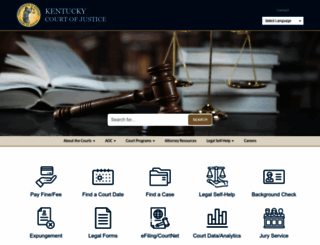A screenshot of the Kentucky Court of Justice webpage showcases a comprehensive user interface designed to facilitate various judicial needs. Dominated by a white background, the page features numerous blue text boxes and blue-colored icons that serve as navigational aids. Centered at the top is a prominent blue banner, adorned with a brown gavel and open books, evoking a courtroom setting. Below this banner, users will find a variety of actionable options, each represented by distinct icons and labeled with clear, blue text.

Key functionalities include a search filter accompanied by a brown search button, providing easy access to specific information. Users can also find options to pay fines or fees, depicted with a drawn-out figure of a hand holding a card. Navigation is further streamlined with icons such as a calendar for finding court dates, a file icon for locating case information, and individual sections dedicated to Legal Self-Help, Background Checks, Jury Service, Legal Forms, and Court Data Analytics.

Each section is clickable, offering expanded information upon selection. The thoughtful design ensures that users can efficiently access the resources they require, whether they are seeking to pay a fee, find a court date, or retrieve legal documents.